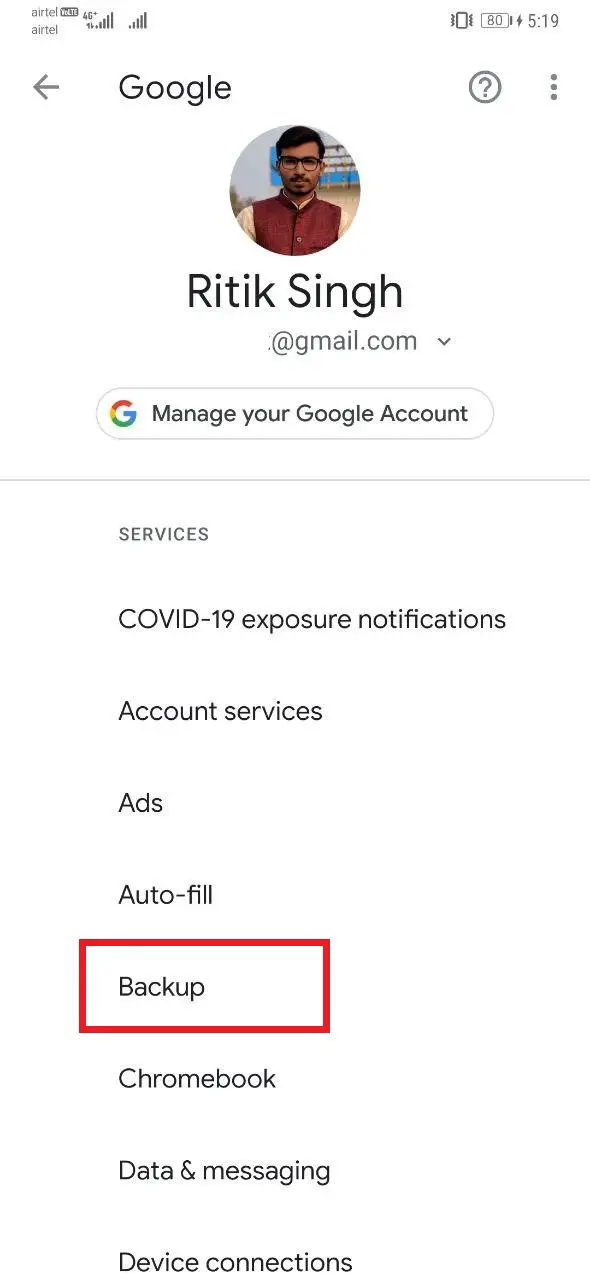Here's the cleaned-up and detailed caption:

---

The screenshot displays various elements of a cell phone's screen, mostly featuring a white background. In the top-left corner, the text "Airtel" is visible twice in black lettering, indicating the service provider. Right next to the second "Airtel" is a rectangular, black and white icon labeled "VoLTE," signifying Voice over LTE support. Adjacent to it are two fully filled internet signal icons.

On the right side of the status bar, the time is shown as "5:19," next to which is a battery icon displaying "80," indicating the battery percentage. The phone's vibration mode is denoted by an icon as well.

Moving down to the left, a black left-pointing arrow is located next to bold black text that reads "Google." Towards the right of this text, there's a white circle with a gray border containing a gray question mark. Further to the right, a vertical ellipsis (three stacked dots) is present.

Centralized below the "Google" label, there’s a profile picture of a man with black hair and glasses, wearing a red shirt with brown sleeves. Beneath the photo, the name "Ritik Singh" is written in bold black letters, with "Singh" as the last name. Below his name, his email address is displayed, featuring a drop-down arrow.

Under this, a white tab with the Google "G" logo on the left side contains the text "Manage your Google Account" in black font. A thick black line separates this section from the settings below.

Starting slightly in from the left, under this line of code, various service options are listed in black text as follows: "Services," "COVID-19 Exposure Notifications," "Account settings," "Ads," "Autofill," "Backup" (outlined in a red rectangle), "Chromebook," "Data & messaging," and "Device connections."

---

This caption provides a detailed and structured description of the elements present in the phone screenshot.